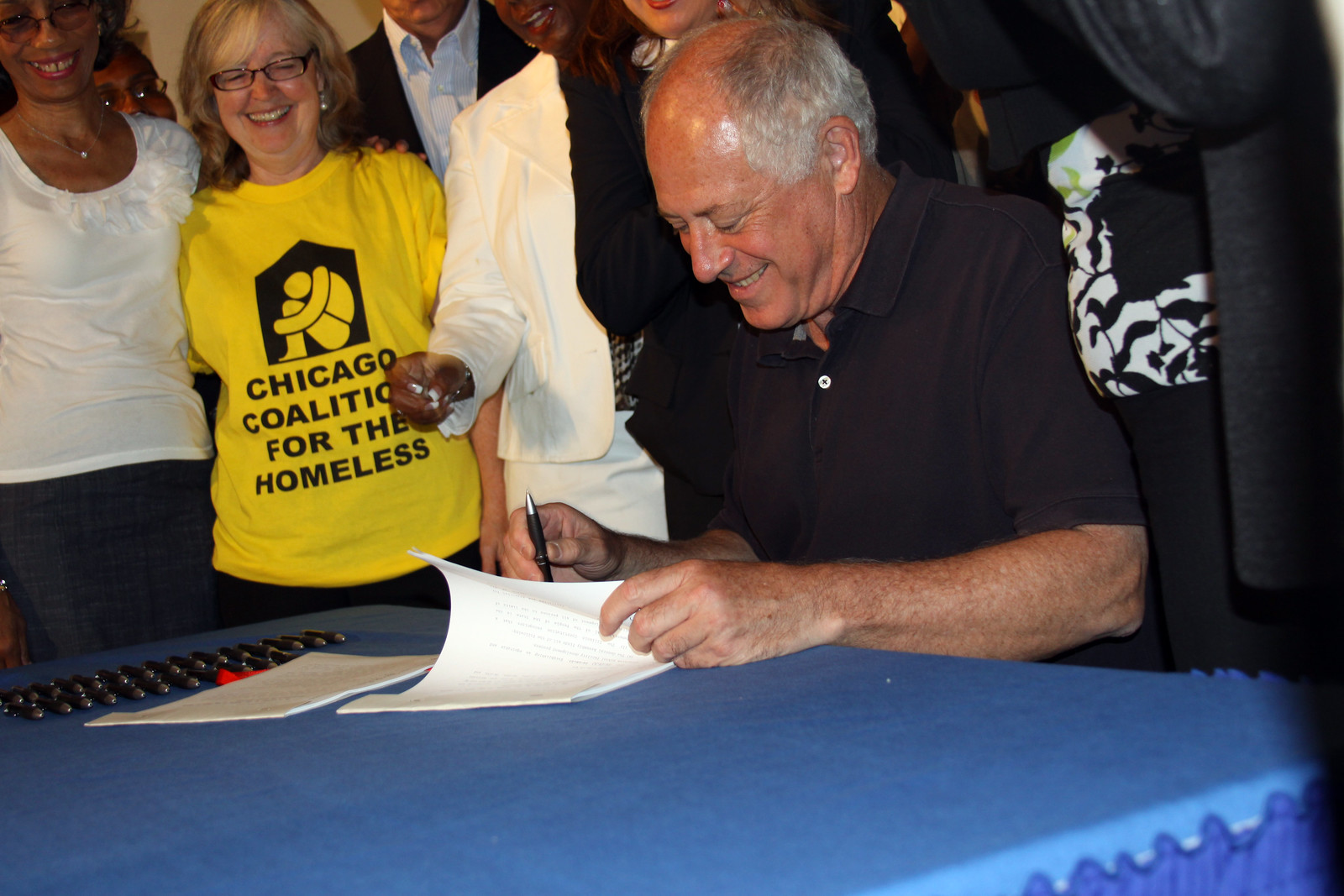In the image, we see an elderly man, likely in his 70s, seated at a table with a blue tablecloth. He’s wearing a short-sleeved black polo shirt, has gray hair, and appears to be signing or reviewing a stack of papers with multiple pens scattered on the table. The man is smiling, fully engaged in the task at hand. Surrounding him are several people, all of whom are smiling and appear to be in a cheerful, supportive mood. A notable woman in a yellow crew neck t-shirt, which bears the logo and text of the "Chicago Coalition for the Homeless," stands closely behind him, smiling. She is a white, chubby woman with glasses and blonde hair. Next to her on her right is an African American woman dressed in a white top and a dark skirt who is also smiling and wearing glasses. Further in the background, a man is seen in a blue-collared shirt with a black suit jacket, partially obscured. Another woman, dressed entirely in white, including a white skirt, is also visible. The scene appears to be joyous, and the man's action might be related to a signing event or another formal acknowledgment, likely organized by the Chicago Coalition for the Homeless.